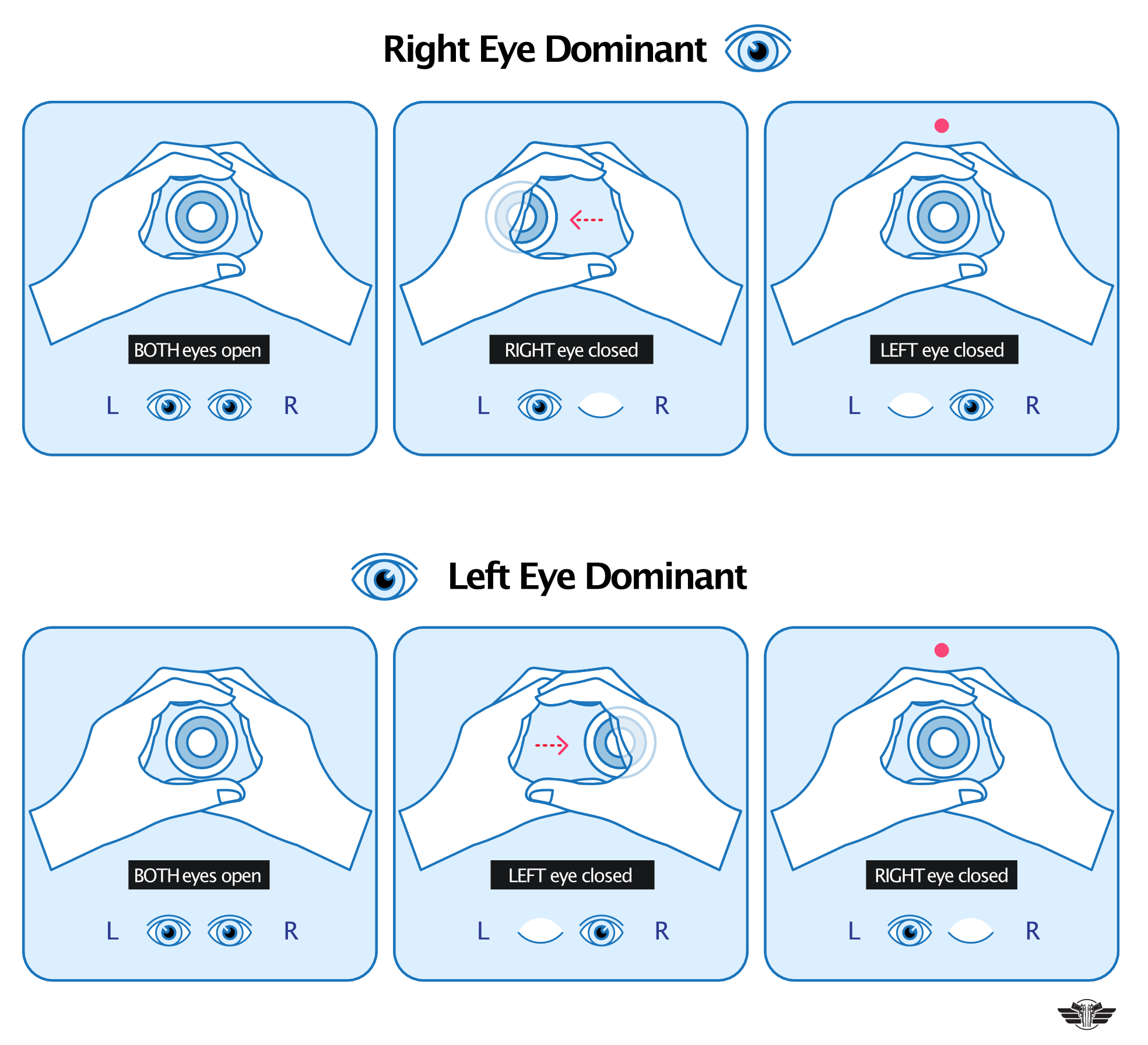The image is an infographic designed to help users determine their eye dominance - whether they are left eye or right eye dominant. It is split into two main sections labeled at the top: "Right Eye Dominant" and "Left Eye Dominant," each containing three distinct diagrams. All diagrams feature a greenish-blue background, with objects in blue or white hues.

In the "Right Eye Dominant" section:
1. The first diagram shows a user with both eyes open, and a target centered between two hands that are cupped around an eye in the foreground, indicating the target is aligned with the user's focal point.
2. In the second diagram, labeled "Right Eye Closed," the target shifts slightly to the left behind the user's left hand, illustrating the view through the left eye only.
3. The third diagram, labeled "Left Eye Closed," shows the target centered within the user's hands again, confirming the right eye is dominant as it remains focused on the target.

In the "Left Eye Dominant" section:
1. The first diagram mirrors the right eye dominant section, with both eyes open and the target centered.
2. The second diagram, labeled "Left Eye Closed," shows the target centered over the right side of the field of view, indicating the view through the right eye.
3. The final diagram, labeled "Right Eye Closed," centers the target again, confirming the left eye's dominance as it remains focused.

At the bottom of the infographic, there is additional explanatory text and visuals, including symbols like "L" for left and "R" for right, and representations of opened and closed eyes corresponding to each exercise. With a focus on hand positioning and target alignment, this infographic offers a detailed guide for users to self-assess their dominant eye through simple exercises.